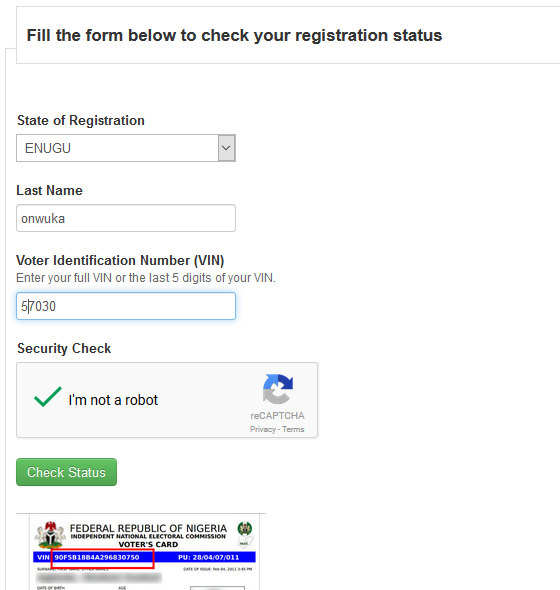The image consists of an online form designed to check voter registration status. The top part of the form resembles a rectangular box, though the right side is cut off. The interior of the box is white, bordered by a gray outline, except on the right side. Bold black text inside the box reads, "Fill the form below to check your registration status."

A thin gray line separates sections of the form. Below this line, the main form area has a white background. The first section is labeled "State of Registration," with both 'S' and 'R' capitalized. This section contains a white rectangular box outlined in gray, filled with the text "ENUGA" in all capital letters.

Following that, there's another section labeled "Last Name," similarly formatted with a white rectangular box outlined in gray, containing the text "ONWUKA." Further down, a section labeled "Voter Identification Number (VIN)" provides instructions in black text: "Enter your full VIN or the last five digits of your VIN." This field is filled in with "57030" and is outlined in blue.

Next, a section titled "Security Check" features a gray box with a green checkmark beside the phrase "I'm not a robot." Additional text in gray reads "reCAPTCHA Privacy - Terms."

At the bottom, there is a green rectangular button with white text that says "Check Status."

The lower segment of the image features a black text block stating, "Federal Republic of Nigeria Independent National Electoral Commission, Voter's Card." It also reveals the voter's VIN number inside a red-bordered box, though the purpose of the red box is unclear.